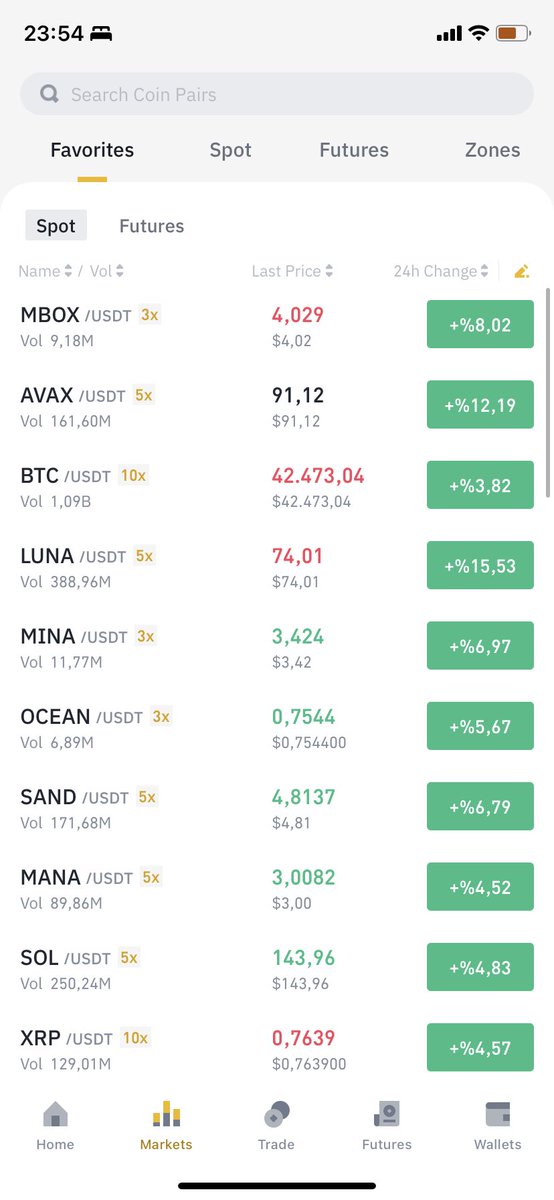The image displays a digital interface, starting at the top left corner with the time "23:54." The battery indicator shows approximately two-thirds charge. Beneath these indicators, there is a search bar, followed by a set of tabs labeled "Favorite," "Spots," "Future," and "Zones" against a light gray background. 

Below this section, the background changes to white, where the tab "Spot" is highlighted. The displayed market data includes:
- "MVOX/USDT 3X" with a volume of "918M," showing a "Last Price" of "4029" and a "24 Hour Change" of "-8.02%."
- "AVAX/USDT" with a volume of "161.60M," showing a "Last Price" of "91.12" with a green background indicating a "24 Hour Change" of "-12.19%."

The interface is organized in columns, with the "Last Price" and "24 Hour Change" columns providing quick reference to the latest trading statistics.